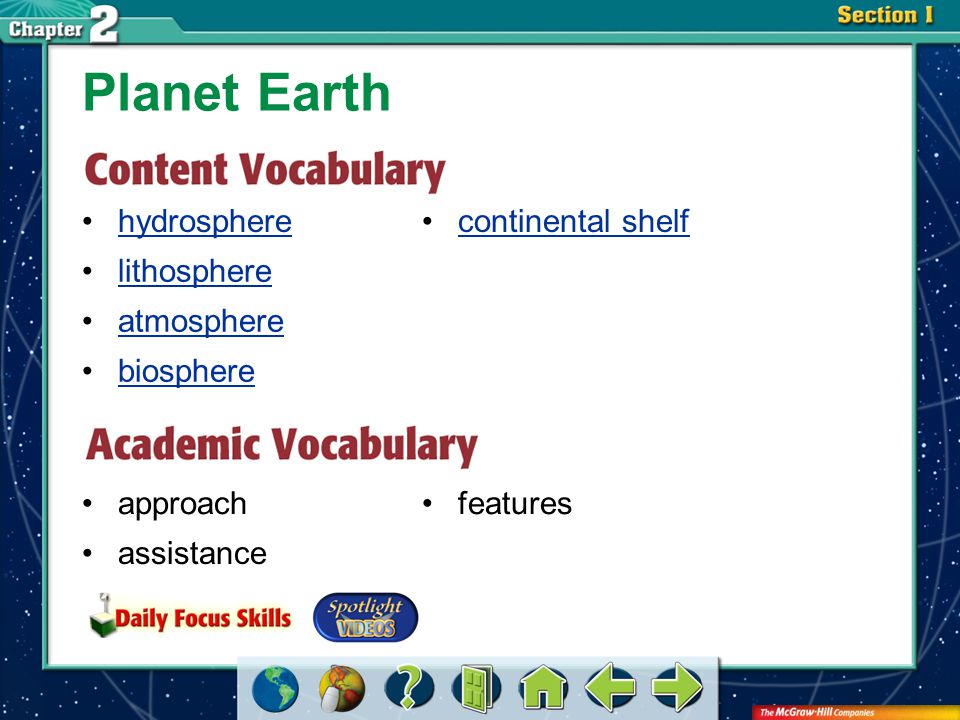The image displays a digital slide or section of a website designed with an educational focus, likely a presentation or online application about Planet Earth. In the top-left corner, white text announces "Chapter 2," while the top-right corner features the yellow text "Section 1." At the center-top of a large rectangular whiteboard area, the green text "Planet Earth" is prominently displayed. Directly below in red text is the heading "Content Vocabulary." Beneath this heading are five blue underlined bullet points: Hydrosphere, Lithosphere, Atmosphere, Biosphere, and Continental Shelf, arranged in a column. To the right, there is another section marked in red text as "Academic Vocabulary," listing three bullet points: Approach, Assistance, and Features. The lower part of the screen includes navigation icons for interacting with the program. Additional elements mentioned are "Daily Focus Skills" and "Spotlight Videos." The visual elements are layered, incorporating a variety of colors including shades of green, blue, white, red, orange, turquoise, burgundy, neon green, beige, and dark blue, adding vibrancy to the educational content.